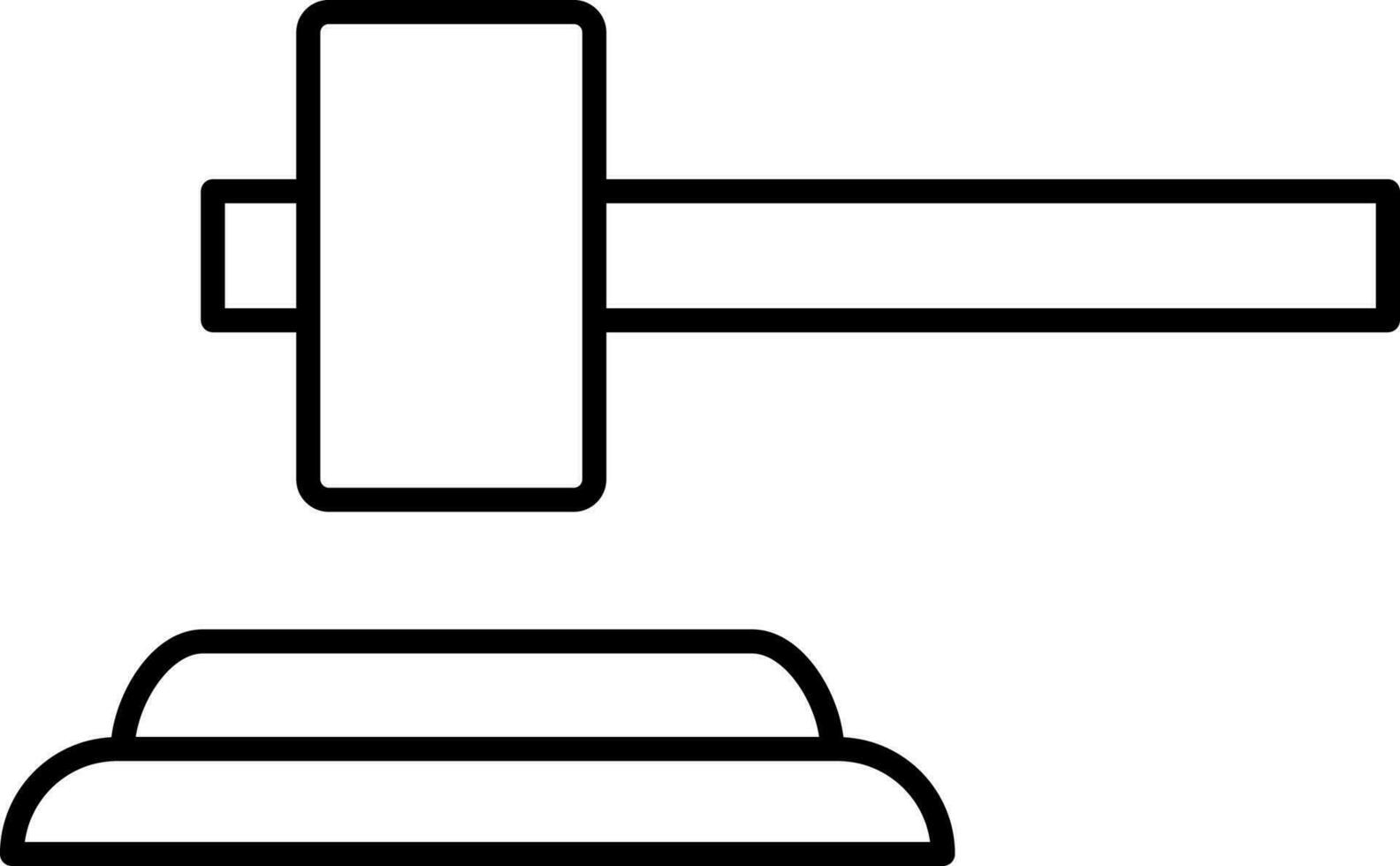The image is set against an all-white background, seamless to the point where the borders of the image are indiscernible, giving it a borderless appearance. The image is oriented in a landscape perspective, being wider than it is tall.

At the center of the composition lies a distinctive illustration of a judge's gavel, which appears to be a modern, stylized interpretation. The gavel's base consists of a two-tiered platform made of wood, where the lower tier is a flat, rounded rectangle which gently curves upward to meet the smaller, flat rectangle on top, creating a stacked effect. 

Situated horizontally above this base is the gavel itself, positioned with its handle facing towards the 9 o'clock direction. The handle, drawn as a long, square-edged rectangle, pierces through the hammer part, which is depicted as a steel, rectangular block rather than the traditional rounded mallet head. This unconventional design gives the appearance of a steel sledgehammer rather than a typical gavel. The overall monochromatic black and white colors add to the stark, minimalist aesthetic of the drawing.